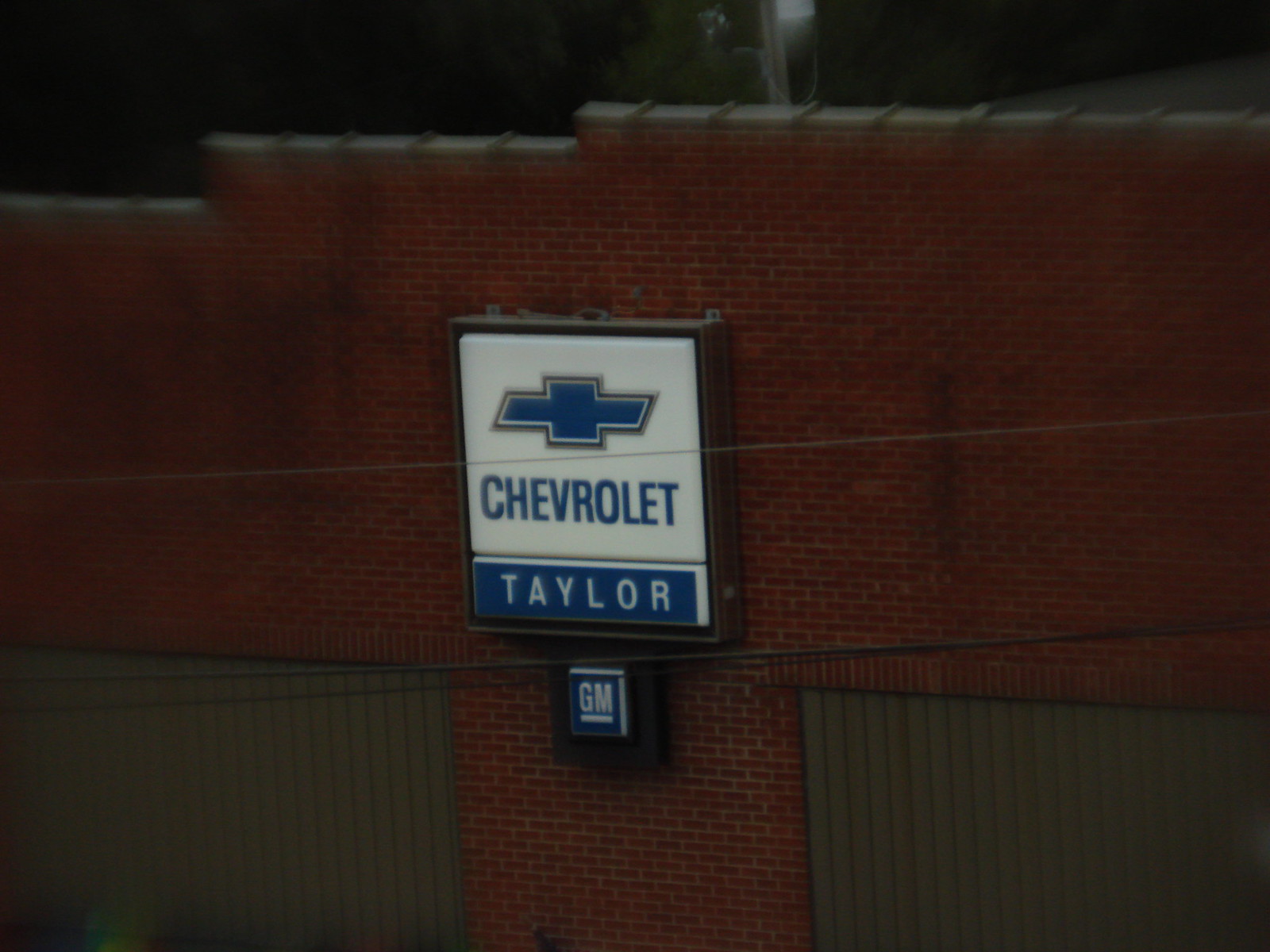In this daytime image, a red brick building stretches upwards as we view it from the ground level. Prominently affixed to the side of the building, just above the first floor, is a square black box sign. This sign, likely illuminated at night, has a white face bearing the iconic blue Chevrolet logo, accented with both black and white outlines. The word "Chevrolet" is boldly displayed in blue letters. At the bottom of the sign, a blue banner features the name "Taylor" in white text. Directly beneath this main sign, there is a smaller rectangular sign displaying the white "GM" logo with an underline. The positioning of these signs is flanked by two olive green closed garage doors, enhancing the old industrial charm of the red brick exterior.